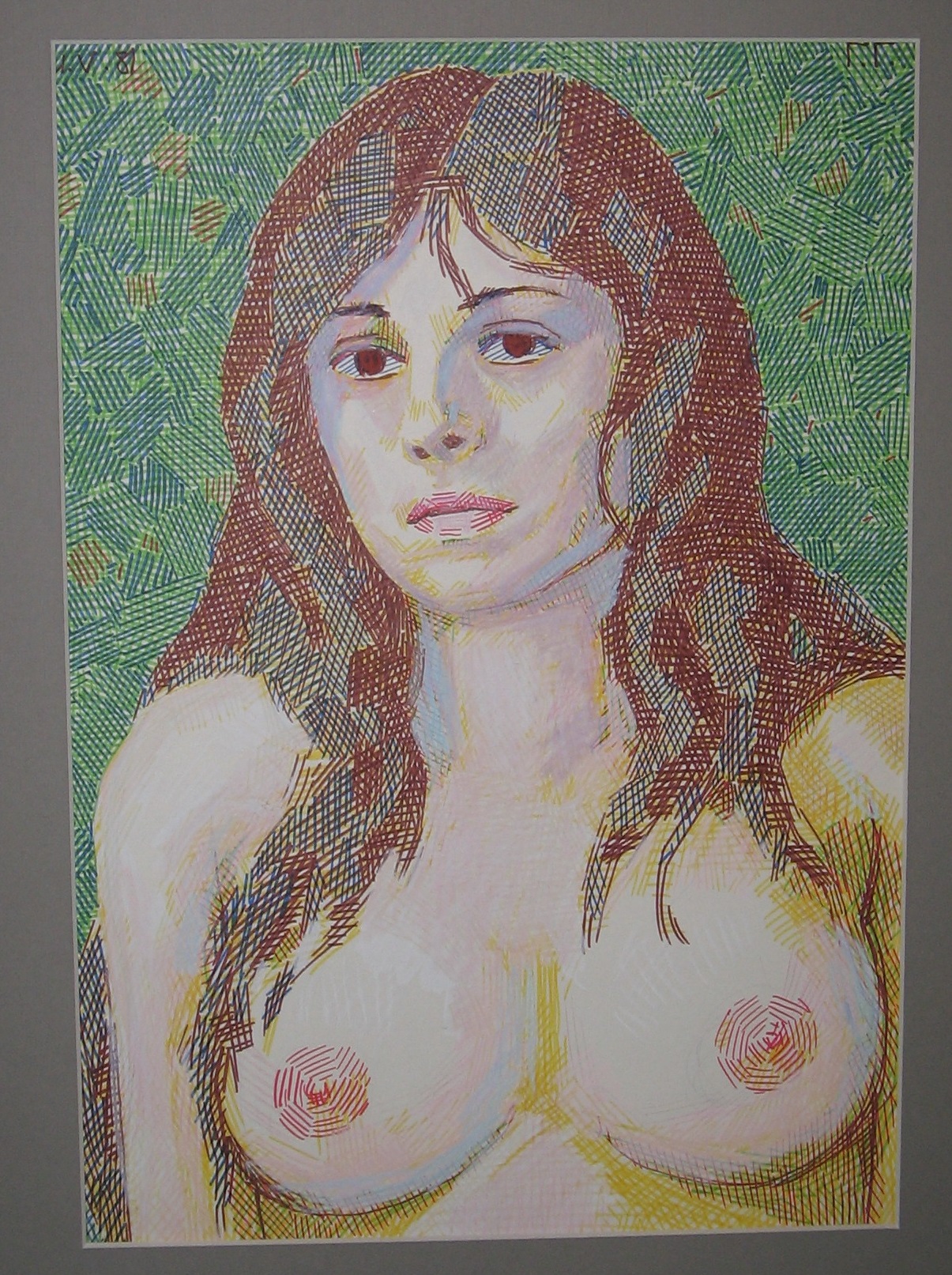This artwork is a detailed drawing of a topless woman with long, wavy brown hair, created through a technique resembling cross-hatching or the use of tiny pencil-like markings. Her hair, accented with subtle green streaks, falls over her shoulders and down her back, with some strands draped across her front. The woman has fair, almost pale skin, brown eyes, and a neutral expression that borders on sadness. Her red nipples are pointed and visibly prominent. The background is predominantly green, interspersed with hints of yellow and orange, providing a subtle contrast to her figure. The overall composition centers around her head, which takes up the top portion of the image, while her torso and arms, with part of her left arm cut off, are positioned below. The image feels like a blend of traditional and pixel art techniques to bring out various shapes and details.